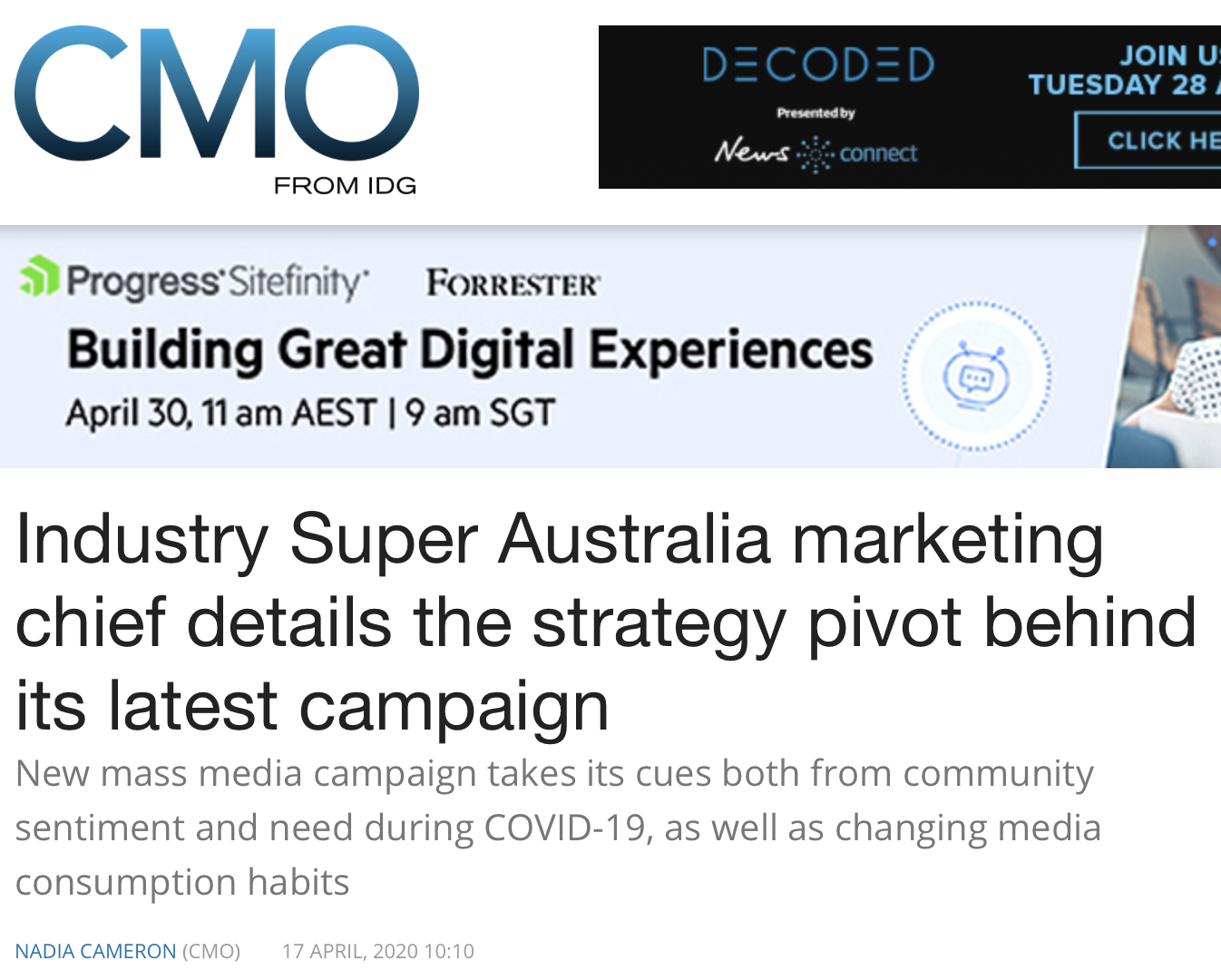In this detailed scene from an industry publication, likely Australian and dated April 17, 2020, several elements catch the eye. The website seems to belong to IDG, a company involved in industry magazines, and prominently features its Chief Marketing Officer. At the top, there are two banner ads, one with a black background and vivid blue text, promoting "Science Decoded" presented by News Connect, inviting viewers to join on Tuesday, the 28th, with a clickable link for more details.

Another banner, on a light blue background, advertises "Progress Sitefinity" in collaboration with Forrester, highlighting their focus on building great digital experiences, with the event set for April 30th. Below these ads, the main article features a piece on "Community Super Australia," where the Marketing Chief outlines the strategic pivot behind their latest campaign. This new mass media campaign is designed to resonate with community sentiment and address needs arising during COVID-19, while also adapting to changing media consumption habits. The article, authored by Nadia Cameron, provides in-depth insights about these shifts and strategies, suggesting links to the evolving marketing dynamics in Australia.